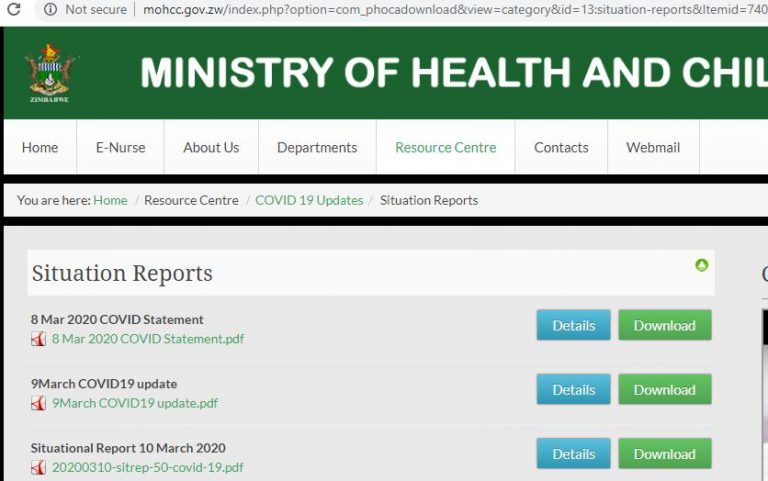The image depicts a blurred screenshot of a website belonging to the Ministry of Health. The URL bar displays a long address, ending with parameters that appear to be related to COVID-19 situation reports. 

The visible portion of the webpage features a navigation bar with menu items including "Home," "eNurse," "About Us," "Departments," "Resource Center," and "Contacts." Below the navigation bar, the user is currently in the "Resource Center" section, looking at the "COVID-19 Update Situation Reports." 

The page lists several PDF documents, arranged by date, with titles such as "8th of March, 2020, COVID Statement" and "9th of March, 2020, COVID-19 Update." Each document entry has buttons labeled "Details" and "Download," with the "Details" button in blue and the "Download" button in green.

The entire image is notably out of focus, making specific text difficult to read. Despite the poor image quality, it's clearly a webpage designed to provide COVID-19 updates and reports to users.